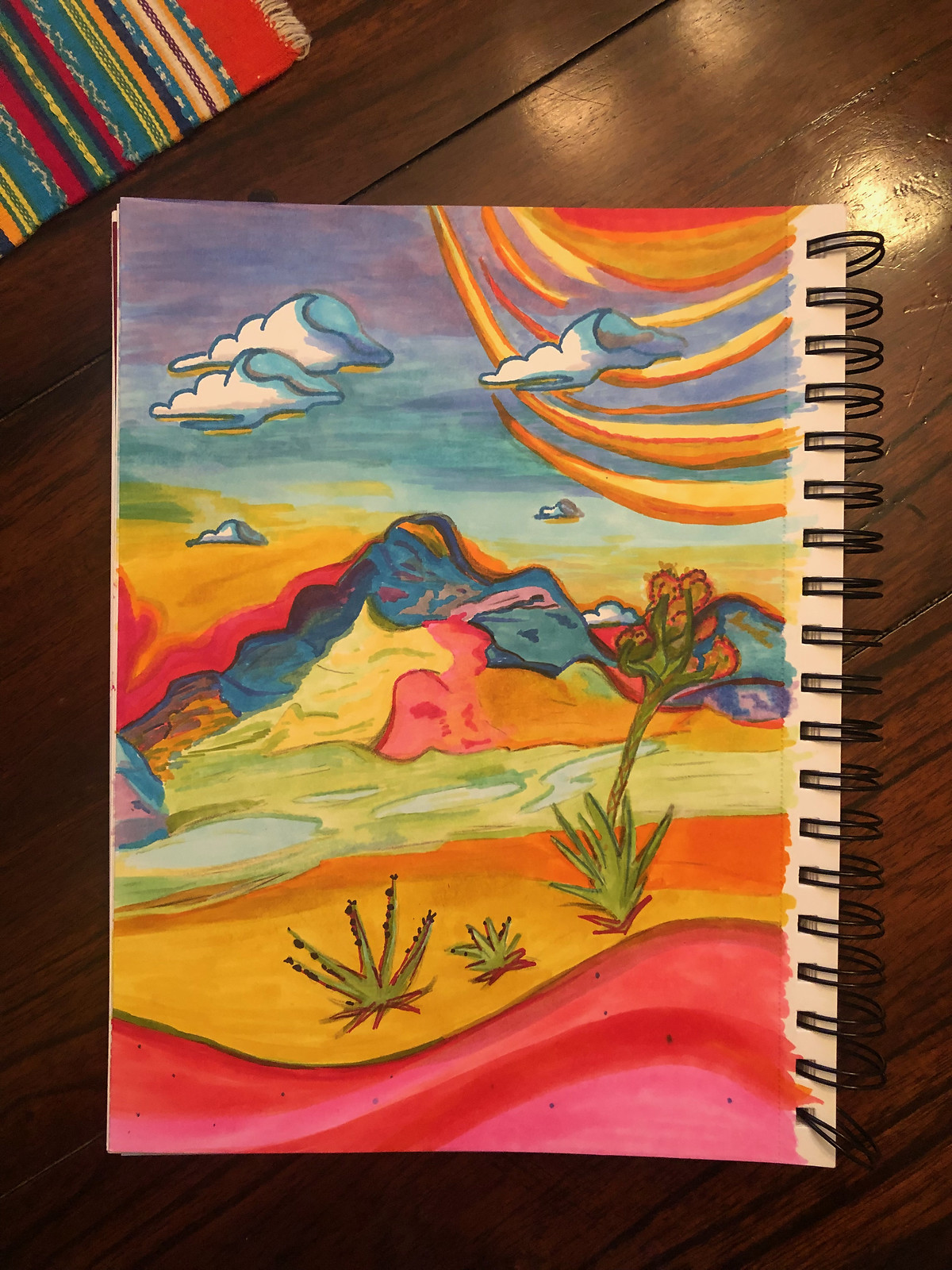On one page of a spiral-wound notebook, there's a distinct and colorful drawing that captures attention with its vivid depiction of a desert scene. The notebook paper, which lacks any clues to indicate its exact size such as 8.5 by 11 or otherwise, is a tan or cream color. The artwork showcases an imaginative landscape filled with exaggerated and vibrant hues, creating an almost surreal environment.

In the mid-foreground, three yucca plants stand prominent, rooted in a striking patch of orange ground. The terrain is a mesmerizing mélange of organic, swooping curves that sweep across the width of the paper, each band noticeably more vivid and saturated than typical natural colors. These bands transition from pink to various shades of red, to a spectrum of oranges, and finally to green interspersed with blue puddles, potentially indicative of rocks rather than water, considering the desert theme.

The background reveals a jagged hill or mountain, constructed from an eclectic mix of amplified colors: bright oranges, greens, dark grays, purples, blues, and yellows merge together to form this striking geological feature. The horizon behind the mountain is awash in the same yellowish-orange hue found near the yucca plants, suggesting a cohesive, fiery desert palette.

In the upper right-hand corner of the sky, a sun is depicted uniquely, surrounded not by conventional rays but by concentric arcs of color. This creative interpretation adds to the otherworldly feel of the scene. The sky itself is a dramatic backdrop of dark tones, dotted with flat-bottomed white fluffy clouds.

This evocative piece of art lies on a wooden table, adding a rustic touch to the setting. In the upper left-hand corner of the notebook page, part of another drawing peeks through, characterized by straight lines of various colors, though it's only a snippet and challenging to decipher its full context.